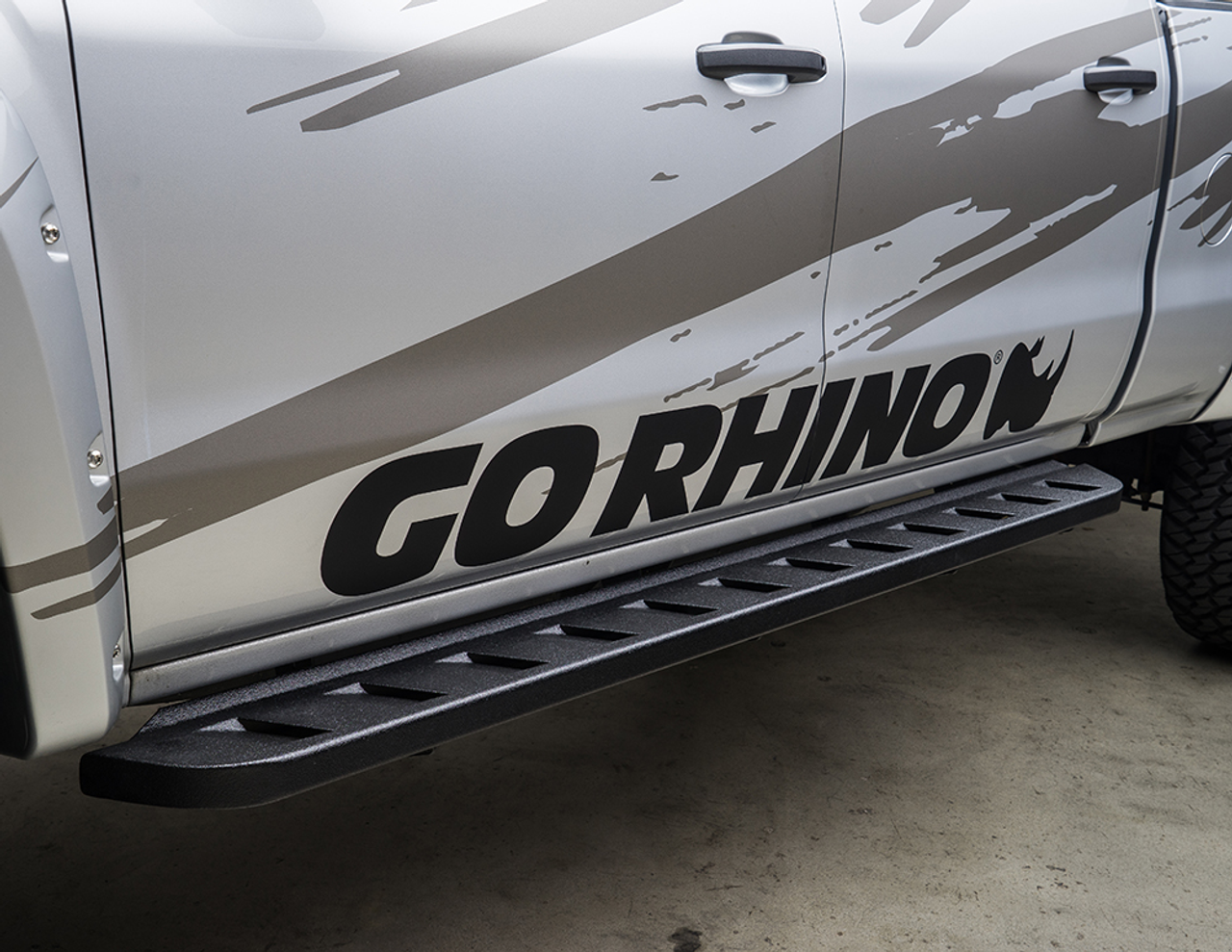The rectangular image, slightly wider than tall, closely captures the side of a double-cabin truck featuring the lower portions of its four doors, with the front and rear doors visible. The truck, positioned at a slight angle, showcases a metallic silvery-white body adorned with diagonal splatter-like streaks of dark tan or gray. Prominently, a black metal footstep runs beneath the doors, descending towards the bottom left corner. The text "Go Rhino" is emblazoned above the footstep, accompanied by a black rhino head logo. Black door handles and the gas tank door further punctuate the truck’s design. The image also includes the front wheel fender and a glimpse of the rear tire, all set against a concrete ground.